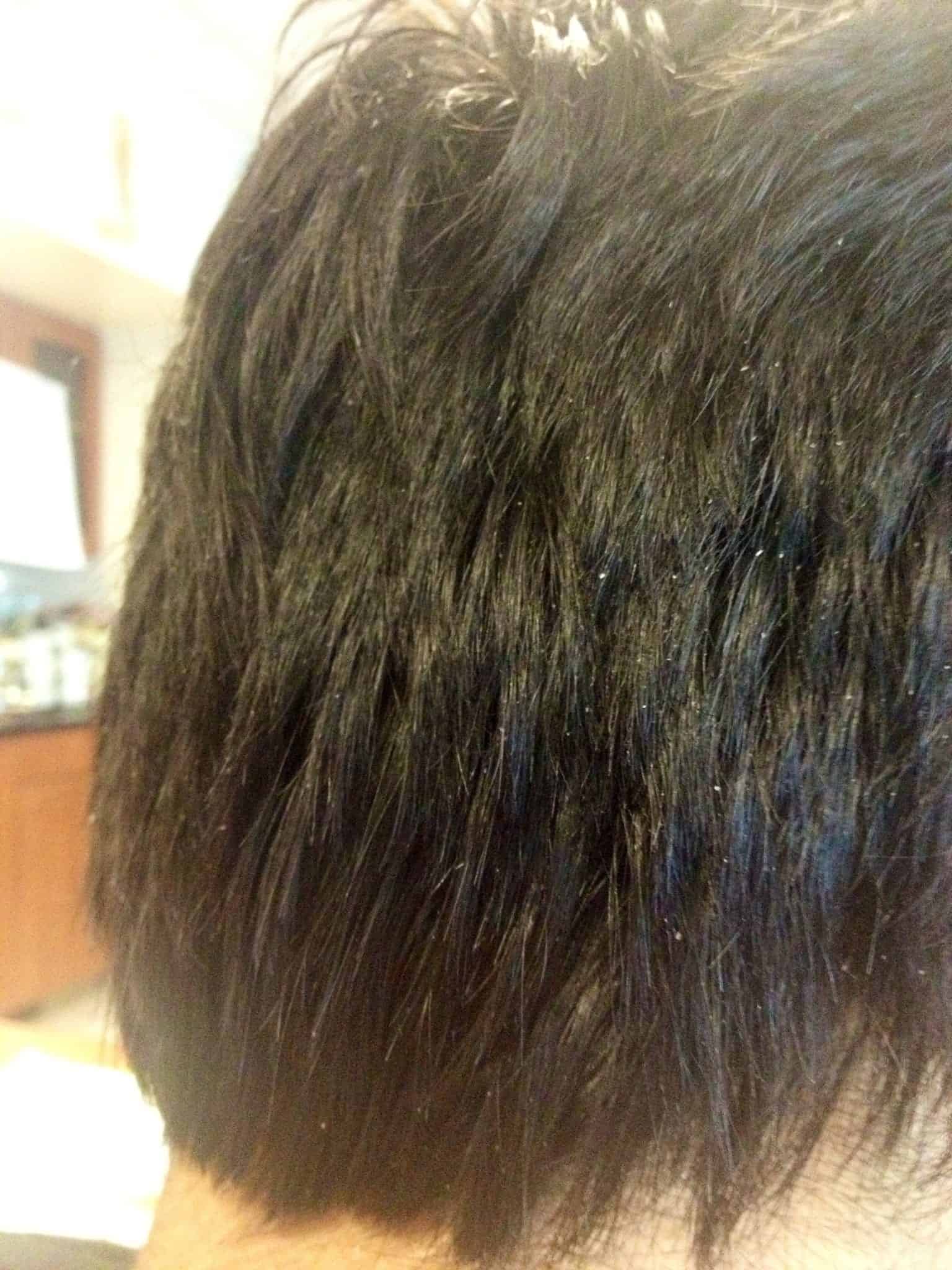The close-up color photograph showcases the back of a Caucasian man's head, focusing on his short, straight, black hair, which is sprinkled with flecks of dandruff. The image includes a bit of his neckline, extending down to the collar of his tan shirt. The upper left corner of the background is illuminated by a bright white light, which fades out some details. Below this light, you can discern a scene consistent with a hair salon or barber shop setting: a wooden cabinet with a black countertop, possibly topped with various bottles; the bottles display mostly white bodies with black and green caps, and a hint of a blue object among them. The white walls and the close-cropped composition of the photograph highlight the dandruff on the man's hair, suggesting it's the primary focus of the image.